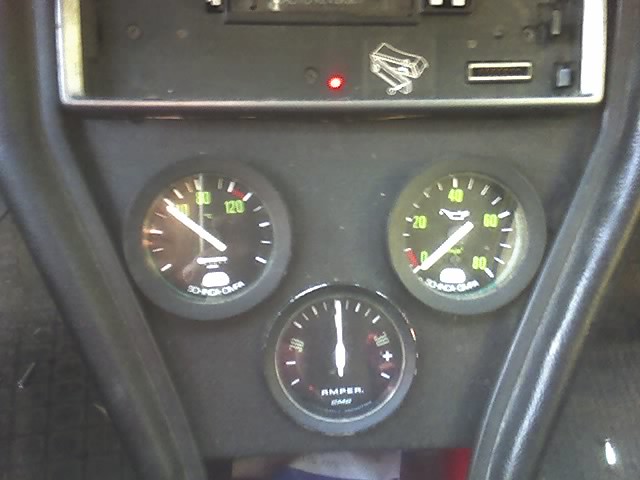The image showcases three analog gauges arranged in a triangular formation against a backdrop of diagonal black lines descending from each top corner. In the upper section, two gauges are positioned side by side, with a third gauge placed directly below them, creating a triangular layout. Above this formation, the bottom half of a metallic rectangle is visible, featuring a red glowing light and some silver rectangular objects.

Each gauge is encased in a circular housing and displays intricate markings. The first gauge on the left has lines encircling its face, with a few numbers present among the markings. The second gauge, immediately to the right of the first, is more detailed, boasting yellow numbers that span its entire circumference. The third gauge, located at the bottom, has fewer numbers, with just two visible on either side. All three gauges are equipped with clock-like pointers indicating various measurements specific to each gauge's function.